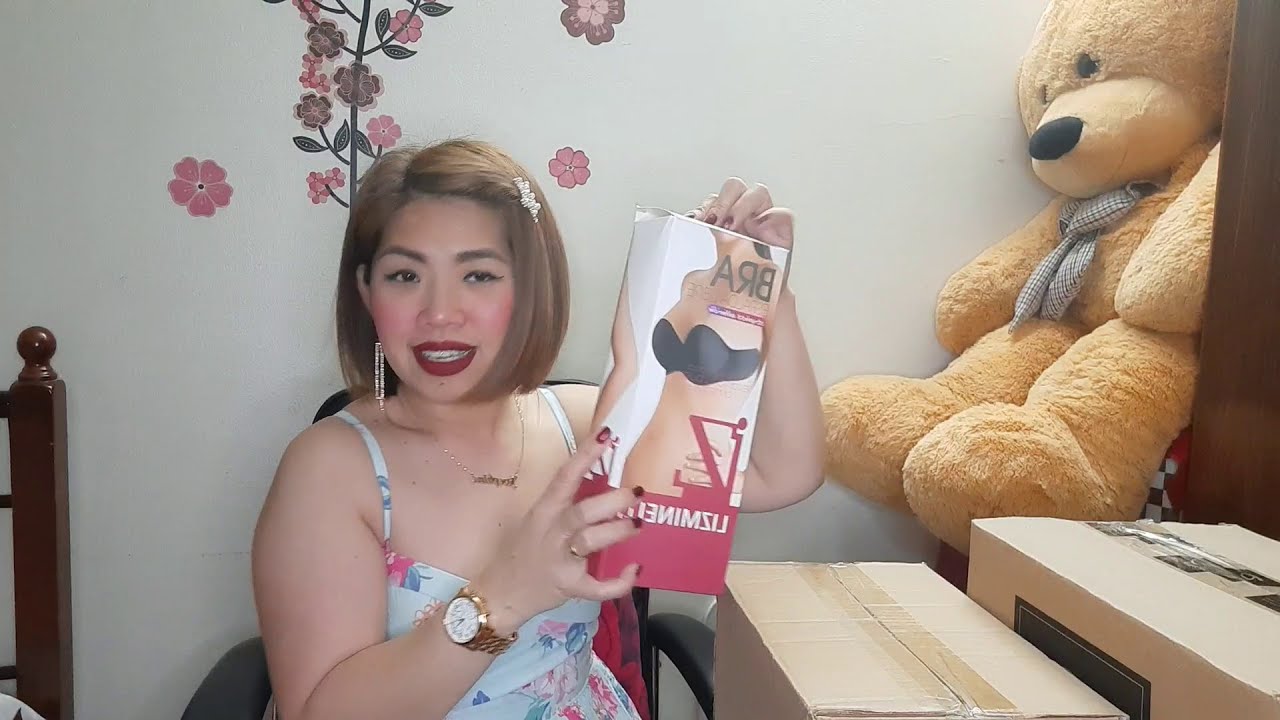The image depicts a young Asian woman with short brown hair styled to her chin and pinned back on one side. She is seated in a chair, possibly streaming a video, as she looks excited and engaged in presenting a product. The woman is holding up a box featuring a black strapless bra, with reversed text beneath the image, indicative of her advertisement or demonstration effort. She is adorned with a necklace displaying her name, earrings, and a gold wristwatch on her right wrist. Her makeup is neatly applied, with deep red lipstick and a pink blush on her cheeks. She's dressed in a floral-patterned blue dress with short sleeves, suggesting a pleasant day.

The background indicates the setting is likely her bedroom. Behind her, the white wall is decorated with pink and green floral wallpaper. On her left is a dark brown wooden bedpost, and on her right, there are several large taped-up cardboard boxes and an enormous light brown teddy bear with a gray accessory around its neck, either a bowtie or scarf. The ambiance is further personalized with other subtle details, including the chair she sits on and the tidy arrangement of her room. Overall, the photograph captures a cheerful moment of the young woman enthusiastically showcasing her recent purchase.